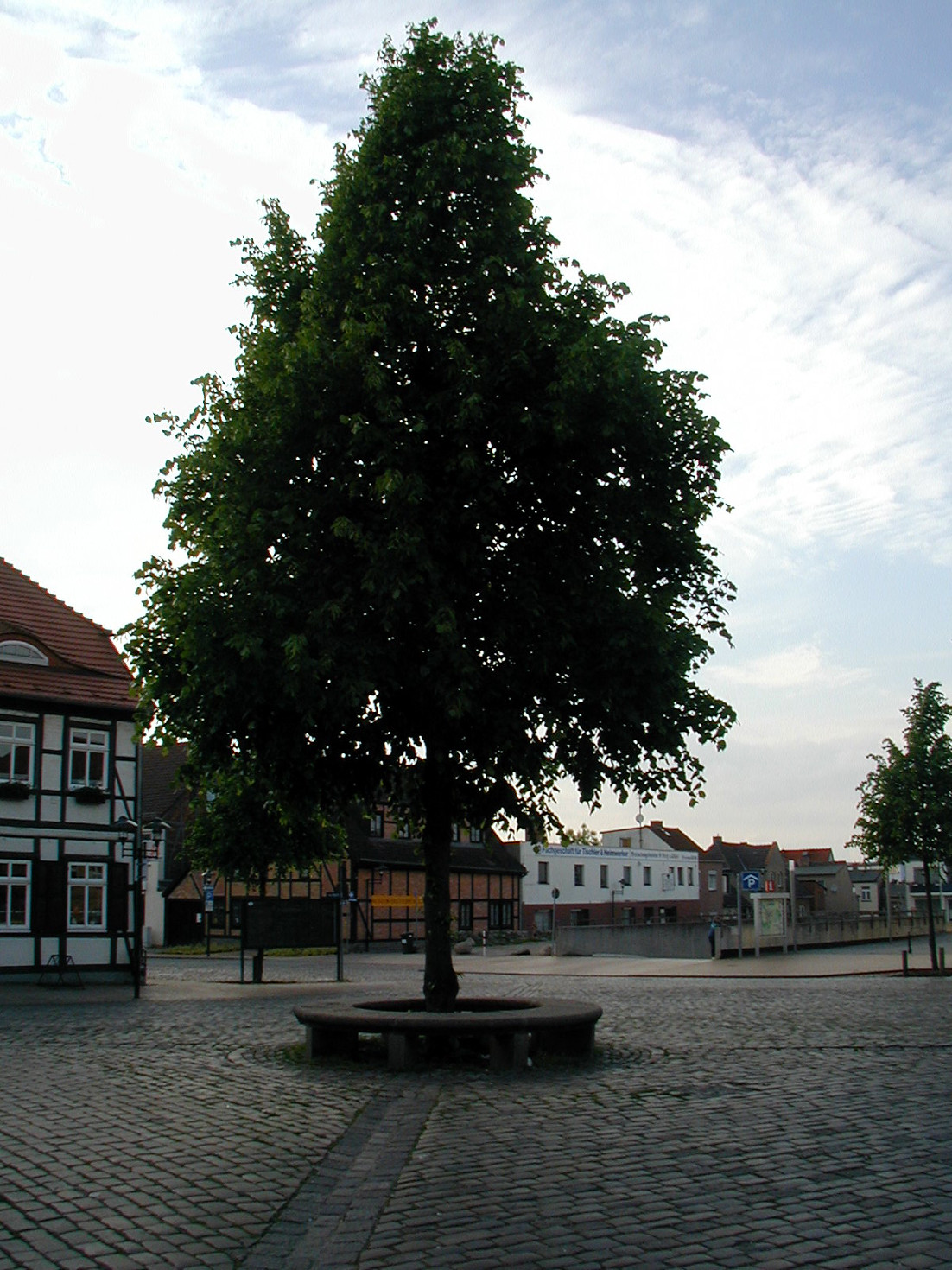A vertical photograph showcases a majestic deciduous tree standing prominently in the middle of a spacious courtyard. The tree, with its lush green foliage and conical shape, towers impressively above the surroundings, reaching nearly three times the height of a nearby two-story house to the left. The courtyard itself is framed by stone walkways, encircling the tree with what appears to be a stone bench, enhancing the impression of a serene, thoughtfully designed urban space. The background features several quaint buildings, likely residential or small shops, emanating a charming, non-commercial architectural style. The partly cloudy sky adds a soft, natural ambiance to the daytime scene, further highlighting the tranquil atmosphere.